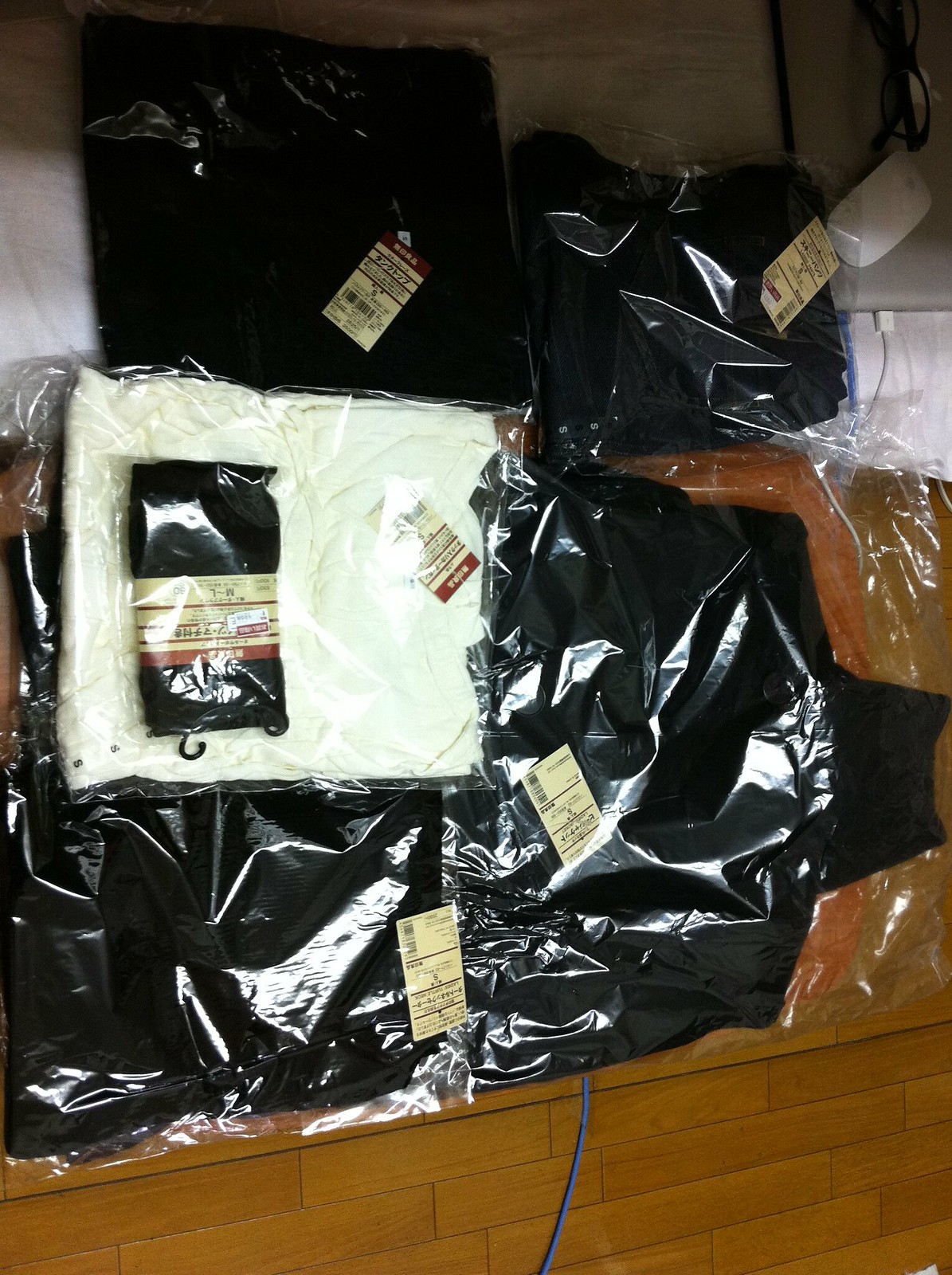The image is a detailed overhead photograph of multiple shrink-wrapped garments placed on a dark brown cherry-paneled wooden floor. In the upper left corner, there is a clear plastic bag containing a black square piece of fabric with a visible tag inside. To the right of this, there is another smaller black piece in a clear plastic bag, also with a tag. Centrally located is a shrink-wrapped white fabric square, topped by a smaller rectangular black item, possibly socks, also in clear plastic with a large tag. Towards the bottom of the photo, there's a large black garment that appears to be a coat or jacket with a turtleneck, shrink-wrapped and tagged. Additionally, in the bottom right corner, a blue ethernet cable is connected to a MacBook, which has an Apple Magic Mouse and a pair of black eyeglasses resting on it, all placed on a white fabric or mattress. The price tags are small and off-white, adding to the sense of a tidy, organized display reminiscent of retail packaging.